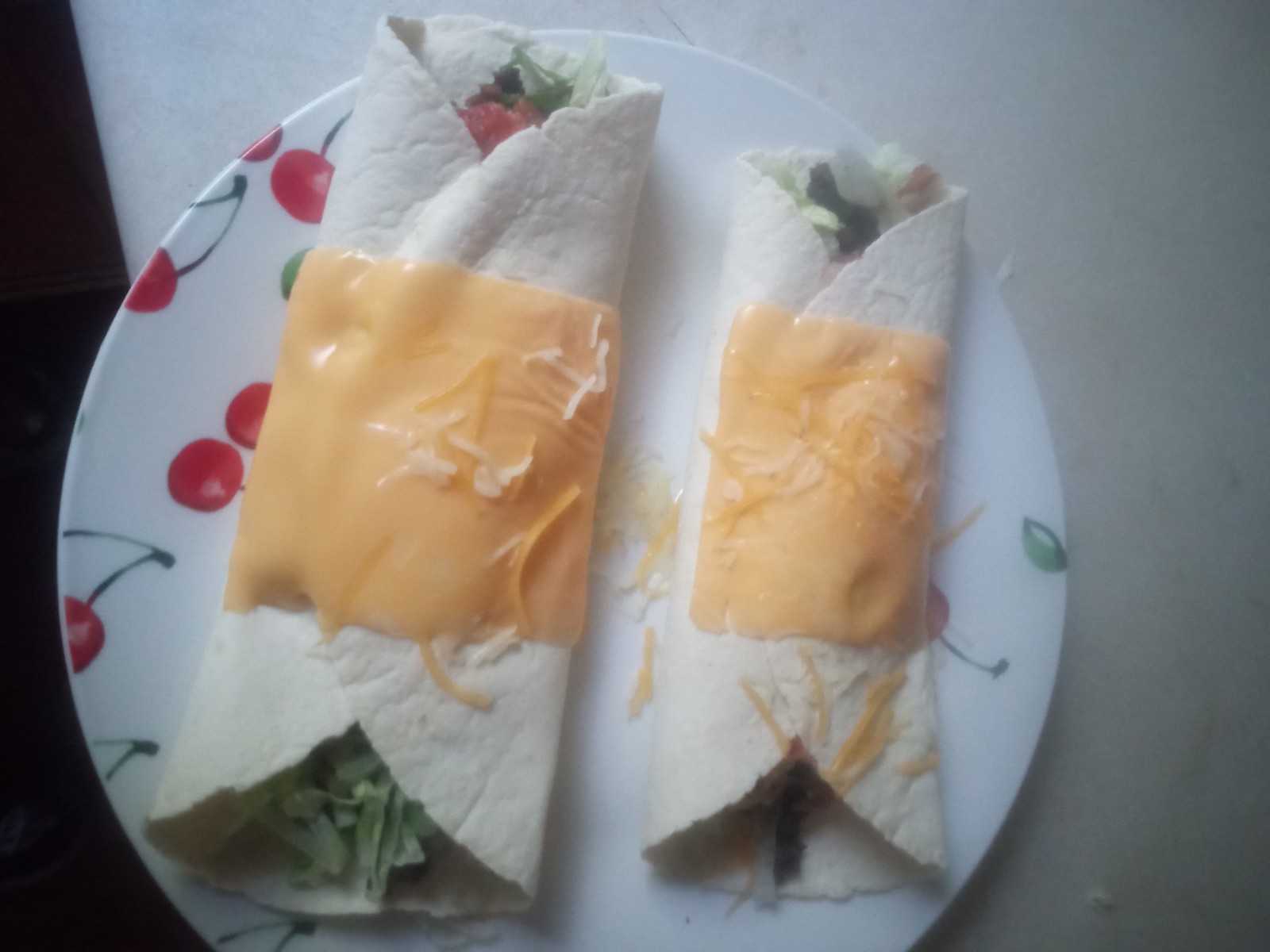In this blurred photograph, likely taken with a phone or an older digital camera considering its hazy quality, two tortilla wraps are centered on a white ceramic plate adorned with scattered red cherries and green stems. The light gray table surface underneath turns a darker gray toward the bottom right of the image. Captured from a top-down perspective, the tortillas are stuffed with mixed salad greens, visibly protruding at both the top and bottom. Each wrap features a slice of melted yellow American cheese, accompanied by shredded cheddar sprinkled over the top, adding a unique texture to the presentation.